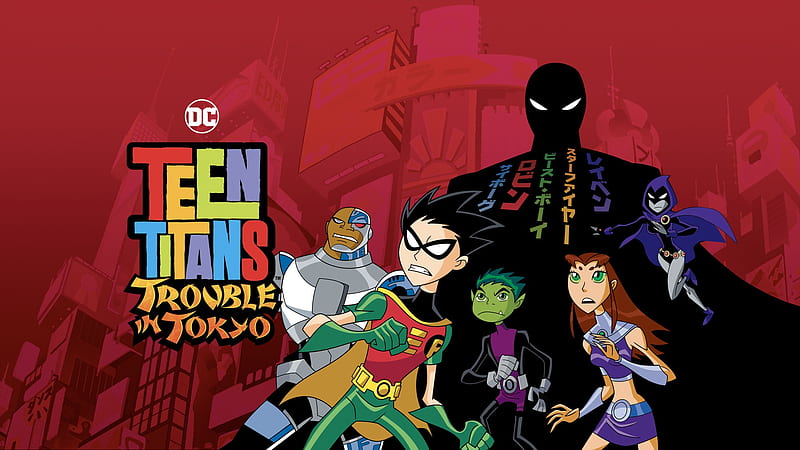The image is a detailed cartoon drawing representing the DC Comics "Teen Titans: Trouble in Tokyo." It features a striking red background that showcases a bustling cityscape with tall buildings. In the foreground, five Teen Titans characters are prominently depicted. At the center is a cybernetic humanoid, half robot and half human, appearing as an African-American male. Next to him stands a fully human character with spiky black hair, a mask, and a costume comprising a black cape with a yellow interior, green gloves, green pants, a yellow belt, and a red top. Adjacent to this character is a boy with green skin and spiky green hair, clad in a black outfit with purple accents. To the right, two female characters with an alien appearance are present. A towering black figure looms in the background, adorned with Japanese characters on his cloak, and ominous white, upturned eyes. The title "Teen Titans: Trouble in Tokyo" is displayed on the left side of the image, anchoring the visual composition.